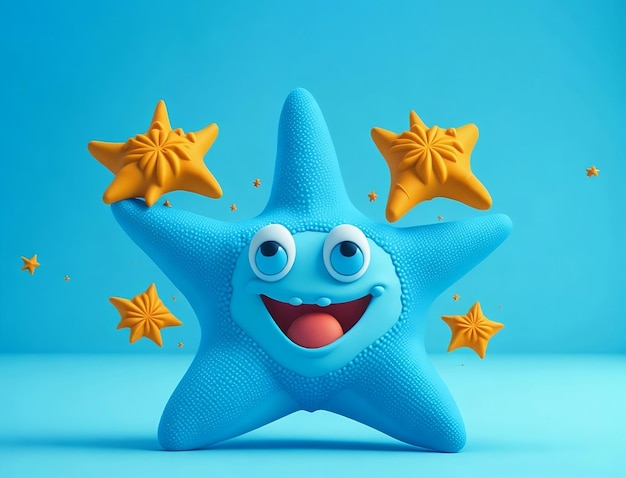The image depicts a computer-generated, cartoon-like blue starfish with prominent facial features. The starfish has large, white eyes with blue centers and small black pupils, along with a wide, smiling mouth that reveals a big red tongue. It appears to be looking up. Surrounding the blue starfish are several yellow stars of varying sizes, which lack facial features and exhibit a secondary star imprinted on them. The background features a gradient of blue shades, with a darker blue occupying the top three-quarters and a lighter blue at the bottom quarter. The overall scene suggests a playful, animated environment, possibly resembling the texture and look of rubber toys.